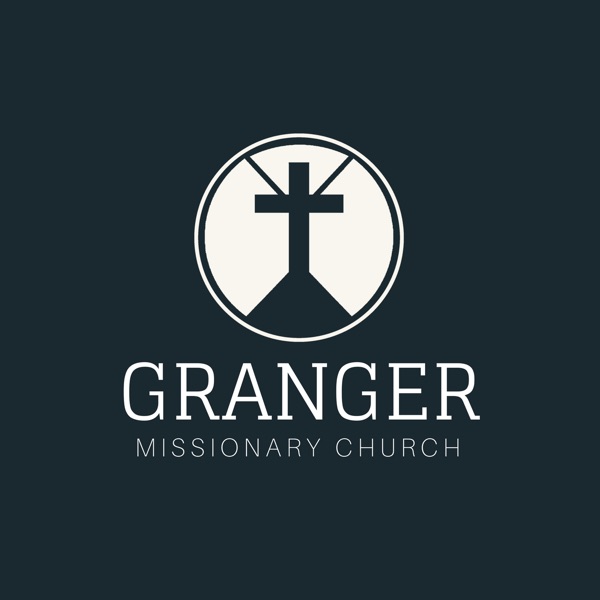The image features a square design with a solid black background. Central to the image is a white circle outlined with a black border. Inside the circle, a black cross is prominently displayed, standing atop a triangular, mountain-like shape. Emerging from the left and right sides of the cross are two angled black lines, forming a V-like configuration. Below the circle, the company name "GRANGER" is written in all caps with white letters, centered directly above the smaller, also all-caps text "MISSIONARY CHURCH," which is similarly in white. The overall composition suggests that this image may be part of a brochure, flyer, or emblem for the Granger Missionary Church.